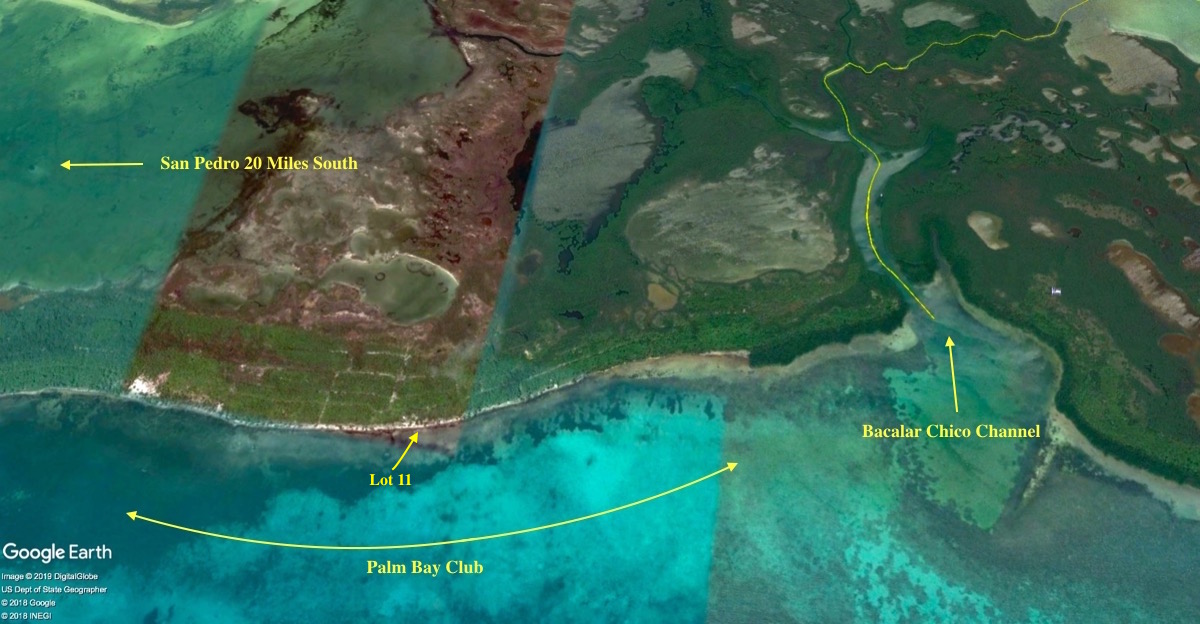The image is a Google Earth snapshot showing the coastal and water regions around San Pedro, Palm Bay Club, and the Bacalar Chico Channel. The map is a horizontally aligned rectangle featuring distinct land and water formations. The left side and upper left corner display greenish-blue water transitioning into land. On the bottom left, it reads "Google Earth," and there’s unreadable smaller print in white. 

Primary details include:
- "San Pedro, 20 miles south," pointed by a thin left arrow in the upper left.
- "Lot 11" marked by a small arrow pointing toward the upper right.
- "Palm Bay Club" indicated by a longer curved line with bidirectional arrows, stretching across the middle portion.
- "Bacalar Chico Channel" in the lower right, denoted by an upward arrow and a channel line extending toward the top right.

The land appears as a mix of marshy terrain and short grassland, garbed with dense trees along the water's edge. Underwater, the right section reveals sand, algae, and potentially coral reefs. Additionally, the top right features sand dunes and varying elevations.